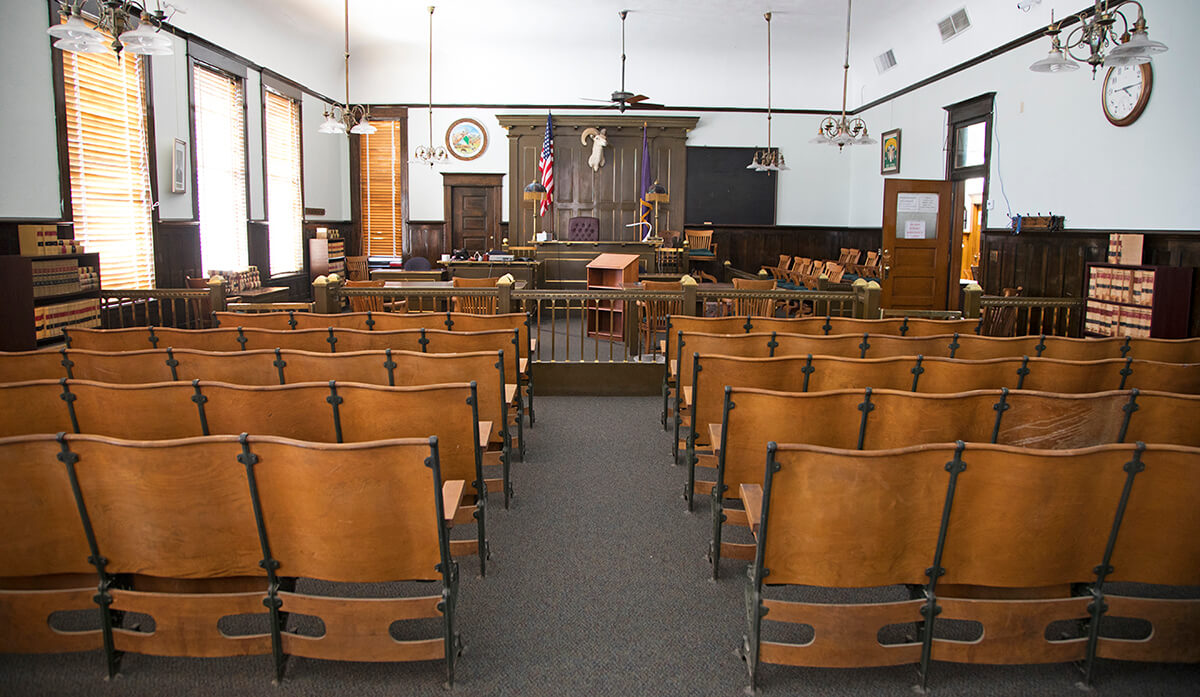This is a detailed photograph of an old-style American courtroom, viewed from the rear as if entering the room. The foreground features several rows of wooden chairs, reminiscent of school seating but without desks, arranged in five rows with an aisle between them. To the left are windows with blinds, while an open door is visible on the right. The room has white walls and a dark grey carpet. A wooden fence runs through the middle, gating off the area where tables and chairs for lawyers are positioned. Beyond this, a slightly raised desk marks the judge's seat, flanked by an American flag on one side and a purple flag on the other. Mounted above the judge's chair is a trophy head of a ram or bighorn sheep. A large clock adorns the right wall. To the far right, there is a section where the jury would sit, further emphasizing the courtroom setting. The courtroom is completely empty, enhancing its historical and solemn atmosphere.